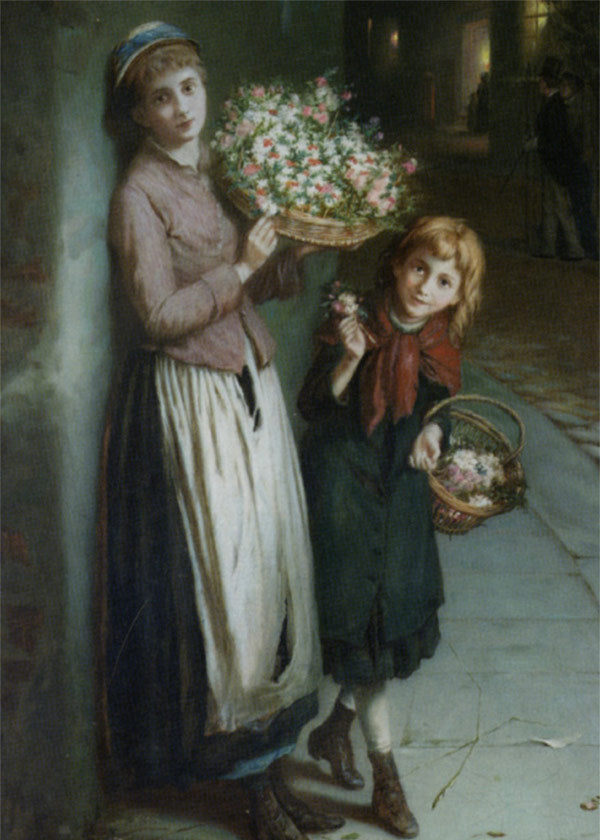The image is a photograph of a late 19th or early 20th-century painting, possibly by an artist like Monet or Degas. It portrays a woman and a young girl, seemingly from the lower Victorian era, engaged in selling flowers. The woman, whose hair is short, is leaning against a concrete wall on an old-time sidewalk strewn with cobblestones. She is clad in a red blouse with a torn white apron atop a blue skirt and a matching blue hat. She's holding up a wicker basket filled with pink and white flowers. 

To her right is a young girl, aged around seven to ten, with red hair and bangs, and a red shawl tied around her shoulders. She wears a blue jacket over a greenish-blue skirt with white stockings and old-timey brown boots. The girl is holding a similar wicker basket containing flowers, its handle strapped over her arm. Both figures appear to be smiling, possibly engaging with the viewer, amidst a backdrop where three finely dressed people walk on cobblestones in the background.